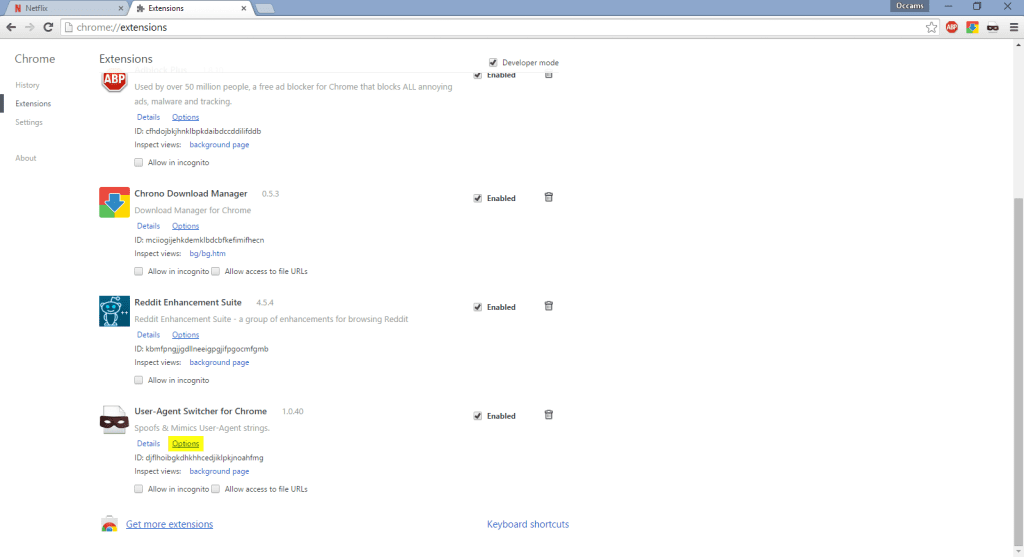The image depicts a web browser window with two open tabs: one for Netflix and another for Chrome Extensions (URL: chrome://extensions). The browser interface shows a navigation pane on the left with options: History, Extensions, Settings, and About Chrome. The 'Extensions' section is highlighted with a black bar.

In the main content area, several Chrome extensions are listed:

1. **Adblock Plus (APB)**
   - Description: "Used by over 50 million people, a free ad blocker for Chrome that blocks all annoying ads, malware, and tracking."
   - Details: 'Details' and 'Options' links are both in blue, with 'Options' underlined.
   - Additional Information: Shows a unique ID number and a blue 'Inspect views: background page' link.
   - Features: Includes an "Allow in Incognito" checkbox, which is currently unchecked.

2. **Chrome Download Manager**
   - Description: "Download Manager for Chrome."
   - Details: 'Details' and 'Options' links are both in blue, with 'Options' underlined.
   - Additional Information: Shows a unique ID number and an 'Inspect views: bg/bg.html' link.
   - Features: Includes checkboxes for "Allow in Incognito" and "Allow access to file URLs," both of which are unchecked.

3. **Reddit Enhancement Suite 4.5.4**
   - Description: "A group of enhancements for browsing Reddit."

Each extension listing includes concise descriptions and various options for further interactions, allowing users to manage their browser extensions effectively.